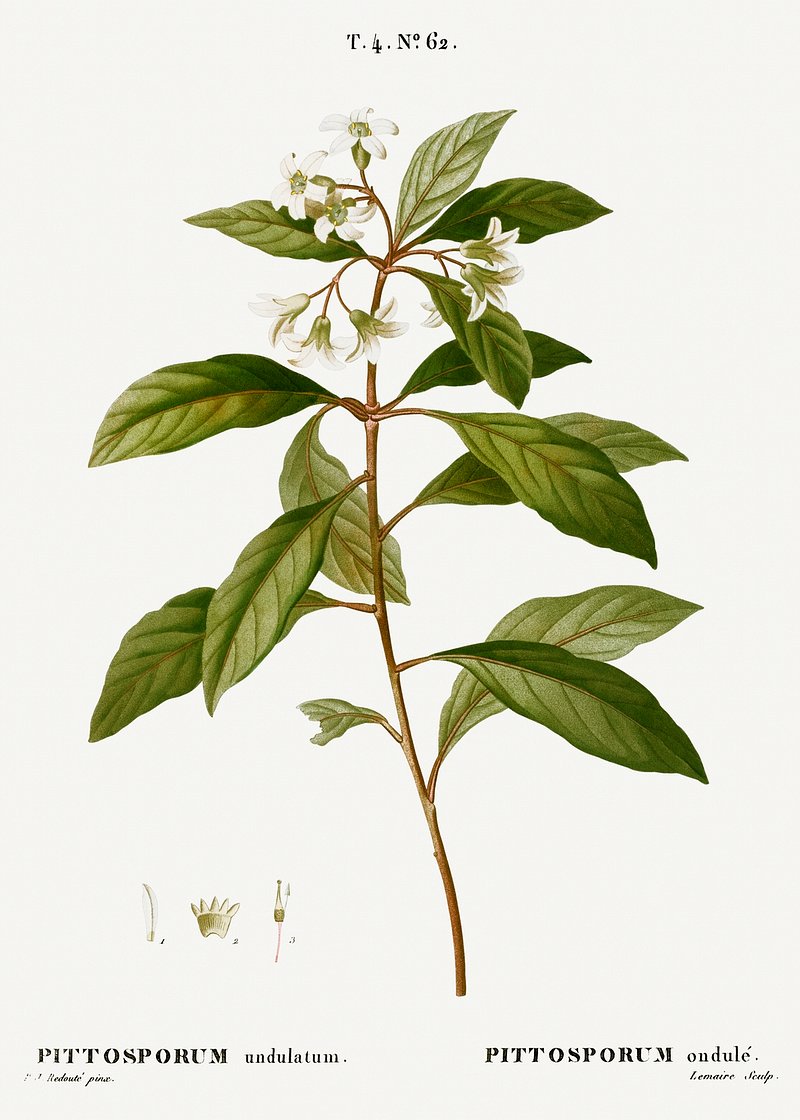This is a colored pencil illustration of a plant known as *Pitosporum undulatum*, depicted with scientific precision. The plant features a tall brown stem that extends upwards, with green, oval-shaped leaves sporadically emerging from both sides. At the apex of the stem, clusters of white flowers bloom. These flowers are bell-shaped with five petals arranged in a circular pattern, encircling a green center and having a green attachment at the back. Some flowers point upwards while others droop downwards. The drawing includes cross-sectional views of different parts of the flower, such as the stamen and ovary, and is set against a white background. Text at the bottom of the image identifies the plant and gives additional scientific information, while the top displays typewritten text including a "T," a "4," and the number "62." This detailed and intricate scientific illustration captures the natural beauty and complexity of the *Pitosporum undulatum*.